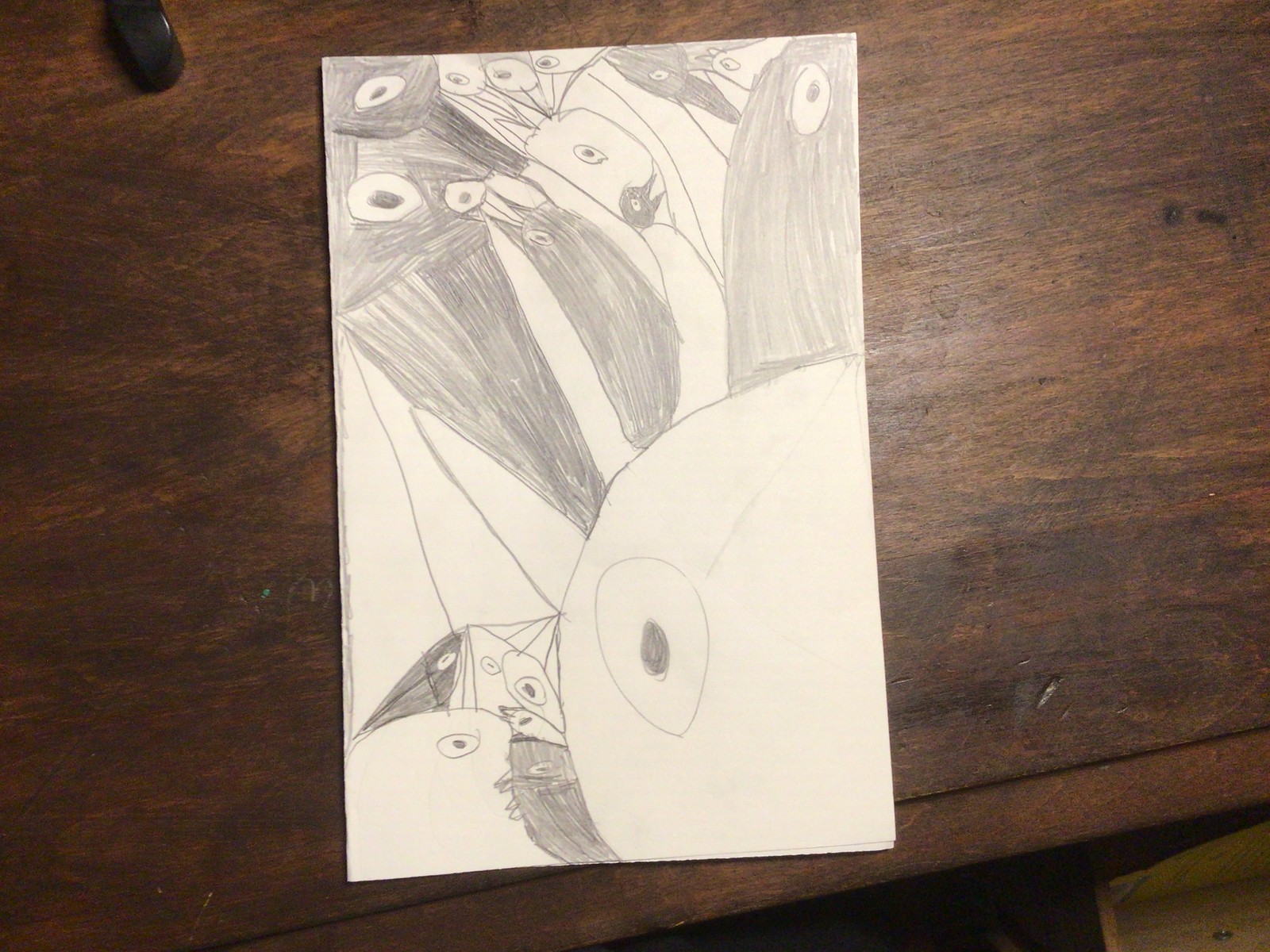On a large, brown wooden table, a black computer mouse rests in the upper-left corner. Beneath the table is a light brown box. In the center of the table lies a large piece of white paper featuring an intricate pencil drawing. The drawing includes a prominent circle in the lower-right corner, within which is a detailed eye—white with a black pupil. The artwork also depicts a small character wearing a dark, pointed hat, with a sharp, pointed face resembling a wolf or coyote. Nearby, a larger character with multiple legs and two large eyes, colored in black, dominates the scene. Additionally, a white dog with a black nose is discernible within the composition.